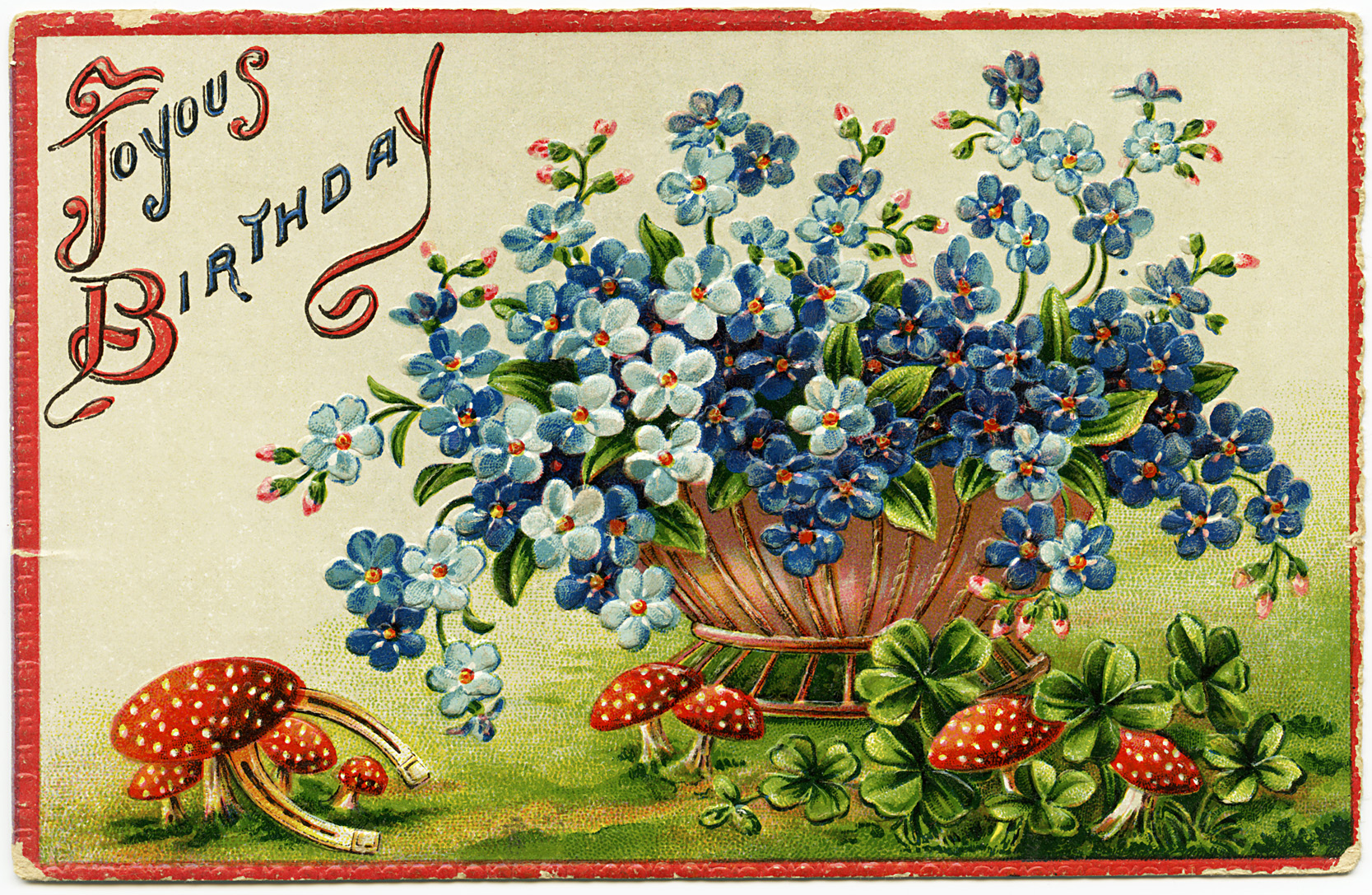This is an illustration designed to resemble an old-fashioned birthday card, hand-painted with meticulous detail. The artwork is framed with a red border that appears intentionally chipped and worn, adding to its vintage charm. In the center of the illustration, a brown planter holds a lush bouquet of blue, light blue, grayish, and white pansies. Interspersed among the flowers are dozens of vibrant red mushrooms with white spots, reminiscent of toadstools or psilocybin mushrooms, hinting at a whimsical or possibly psychedelic undertone. Particularly noticeable are the clusters of red mushrooms growing to the right of the planter and a few on the left, amongst which a golden horseshoe is visibly tucked, symbolizing good luck. Surrounding these elements are lush green shamrocks, prominently featuring four-leaf clovers. The top left corner of the illustration bears the handwritten text "Joyous Birthday" in an old-fashioned font, with "TOYOUS" written as "T-O-Y-O-U-S" in some parts, combining red fancy letters with simpler blue ones. This detailed, high-quality artwork captures a sense of nostalgia and whimsy, making it a captivating depiction.